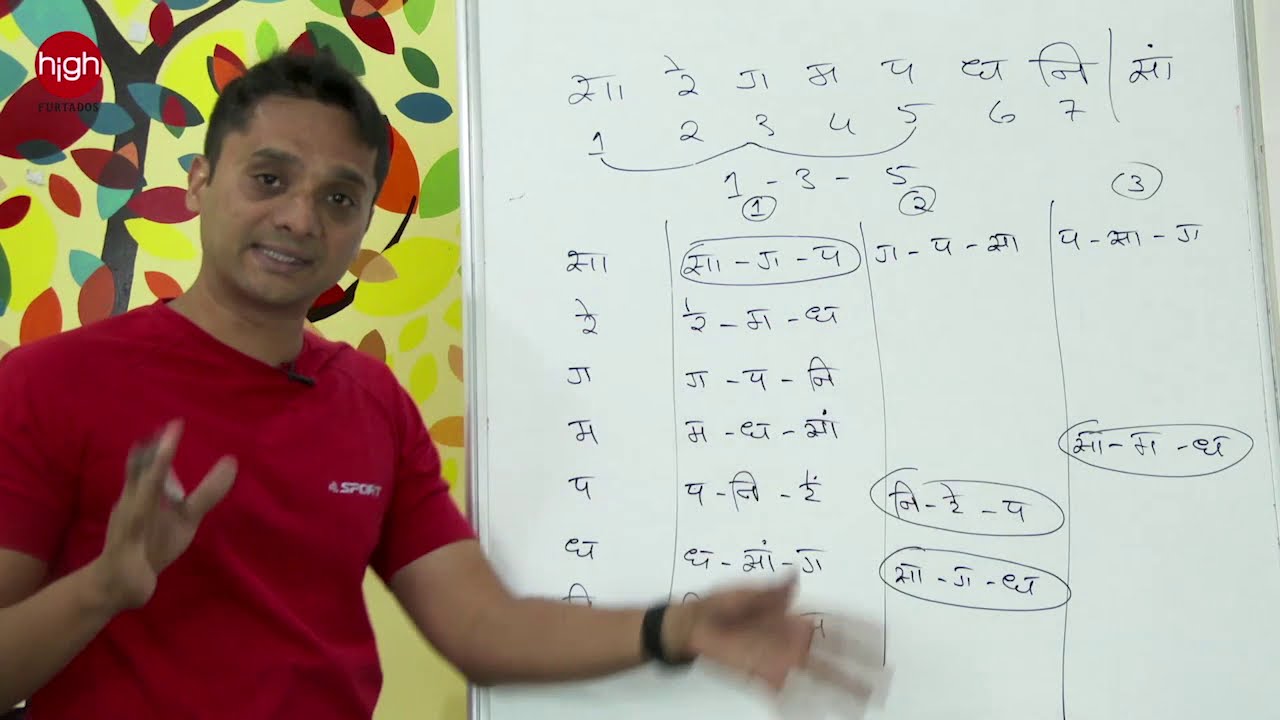In this vibrant and detailed image, an Indian man, presumably a math teacher, is actively engaged in explaining a complex mathematical problem. He stands to the left side of the rectangular frame, wearing a red shirt emblazoned with the word "sport." The man has dark brown or black hair, a tanned complexion, and sports a tiny microphone at his neckline, hinting at an instructional setting. His right elbow is bent with his palm facing forward, and his left arm is slightly extended, likely gesturing to the whiteboard that dominates the center to the right side of the image.

The large whiteboard is covered in a multitude of numbers and symbols, arranged in multiple lanes or rows. Visible figures include sequences like 2, 11, 2, 3, 4, 5, 6, 7, and possibly some fraction marks like "1/2," with certain elements circled, emphasizing particular points in his explanation. He uses a blue or black dry erase marker to write on the board.

Behind the man, stretching across the background on the left, is an eye-catching mural featuring a stylized tree with leaves of various bright colors—red, yellow, blue, green, and orange—contributing to the image's vivid and dynamic atmosphere. Additionally, there's a red circle with the word "hi" in white letters located in the upper left corner of the image, further enhancing the engaging teaching environment. The man also wears a smartwatch with a black band on his left wrist, adding to his modern and professional appearance.